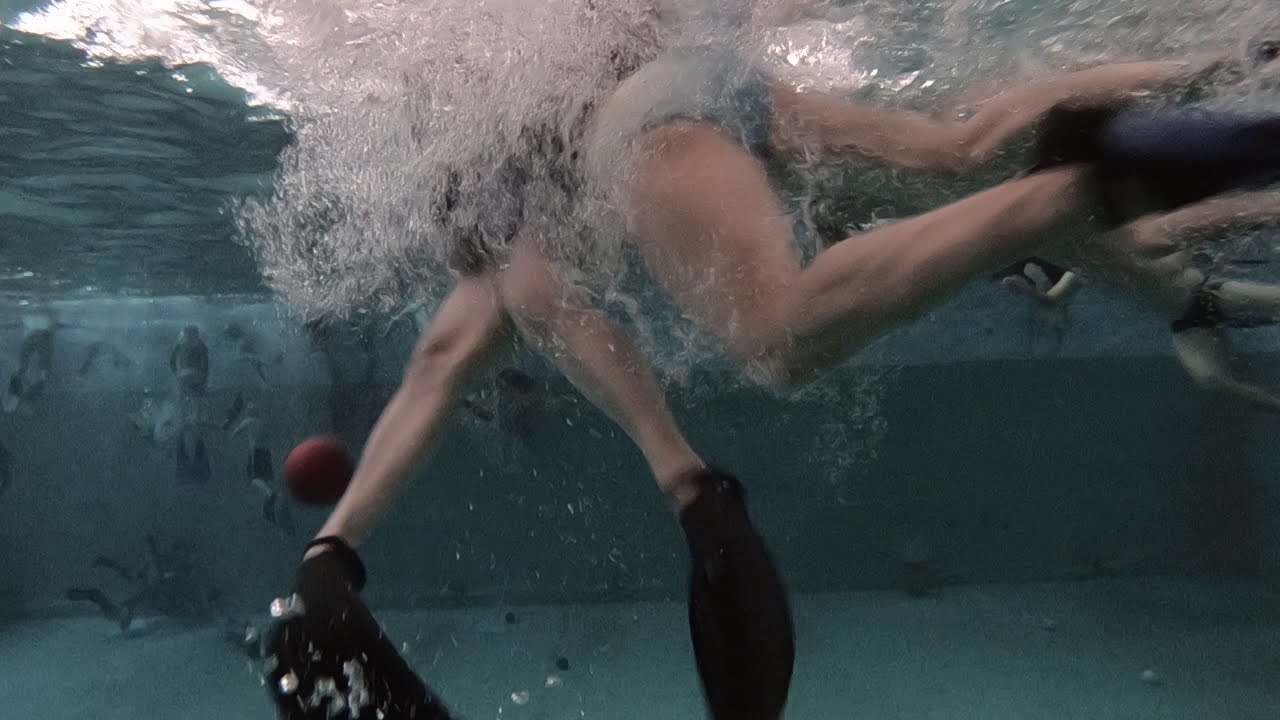This underwater photograph captures an intense moment in a swimming pool, likely during a water sports game. The image, approximately six inches wide by three inches tall, focuses on the legs of several participants. The water is a mix of light blue near the center, darkening to a bluish-gray further out. Bubbles and white turbulent water dominate the upper left corner, indicating lively activity.

Central to the image, we see the backside of a person of Caucasian descent wearing a light blue Speedo and black flippers, seemingly colliding with another individual in a dark swimsuit, also wearing black flippers. Both individuals appear to be of Caucasian descent, and their legs are visible from the knees down.

To the lower left, near one person's leg, a reddish-brown ball can be seen, suggesting the presence of a water polo game or similar sport. Further back, more people equipped with swim trunks and diving flippers are visible, either at the pool's bottom or swimming upward, enhancing the sense of action and competition. The overall atmosphere is dynamic, filled with movement and energy.